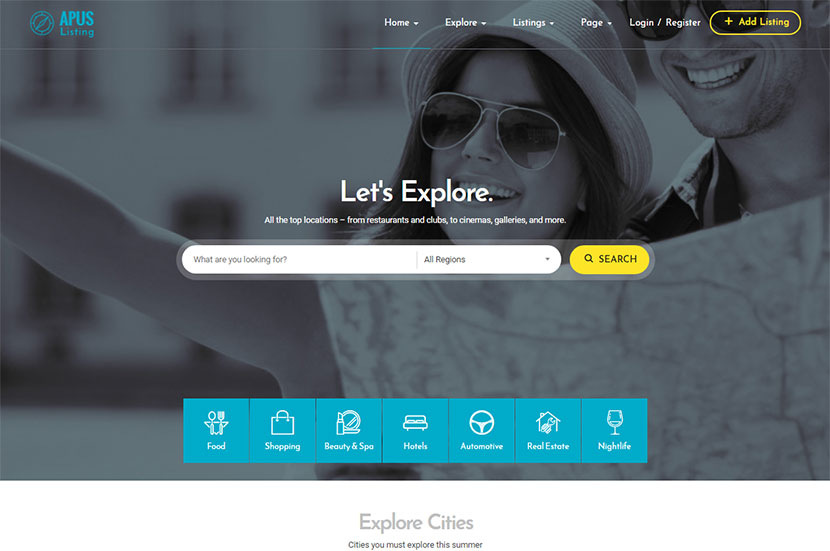A screenshot of the landing page of the website "APIS Listing". In the upper left-hand corner, against a gray background, there's a compass icon with the site's name "APIS Listing" displayed in turquoise lettering to the right of it. On the right-hand side of the page, there's a selection bar with white text options including "Home," "Explore," "Listing," "Page," "Login/Register," and a yellow oval button labeled "Add Listing."

In the center, bold white lettering on the gray overlay states "Let's Explore." Below this, the text reads "All the top locations from restaurants and clubs to cinemas, galleries, and more." Beneath this, there is a white oval text entry field with the prompt "What Are You Looking For?" Adjacent to this, on the right, is a dropdown option labeled "All Regions," next to which is a yellow oval button for submitting the search.

A turquoise bar spans the bottom of the page, featuring seven icons labeled from left to right: "Food," "Shopping," "Beauty and Spa," "Hotel," "Automotive," "Real Estate," and "Nightlife." At the very bottom, in gray text, it reads "Explore Cities," with a black subheading stating "Cities You Must Explore This Summer."

The background image, behind all the text and interactive elements, shows a young couple. On the right-hand side of the image, they are holding up a map and appear to be tourists, complete with sunglasses, a sun hat, and big smiles.